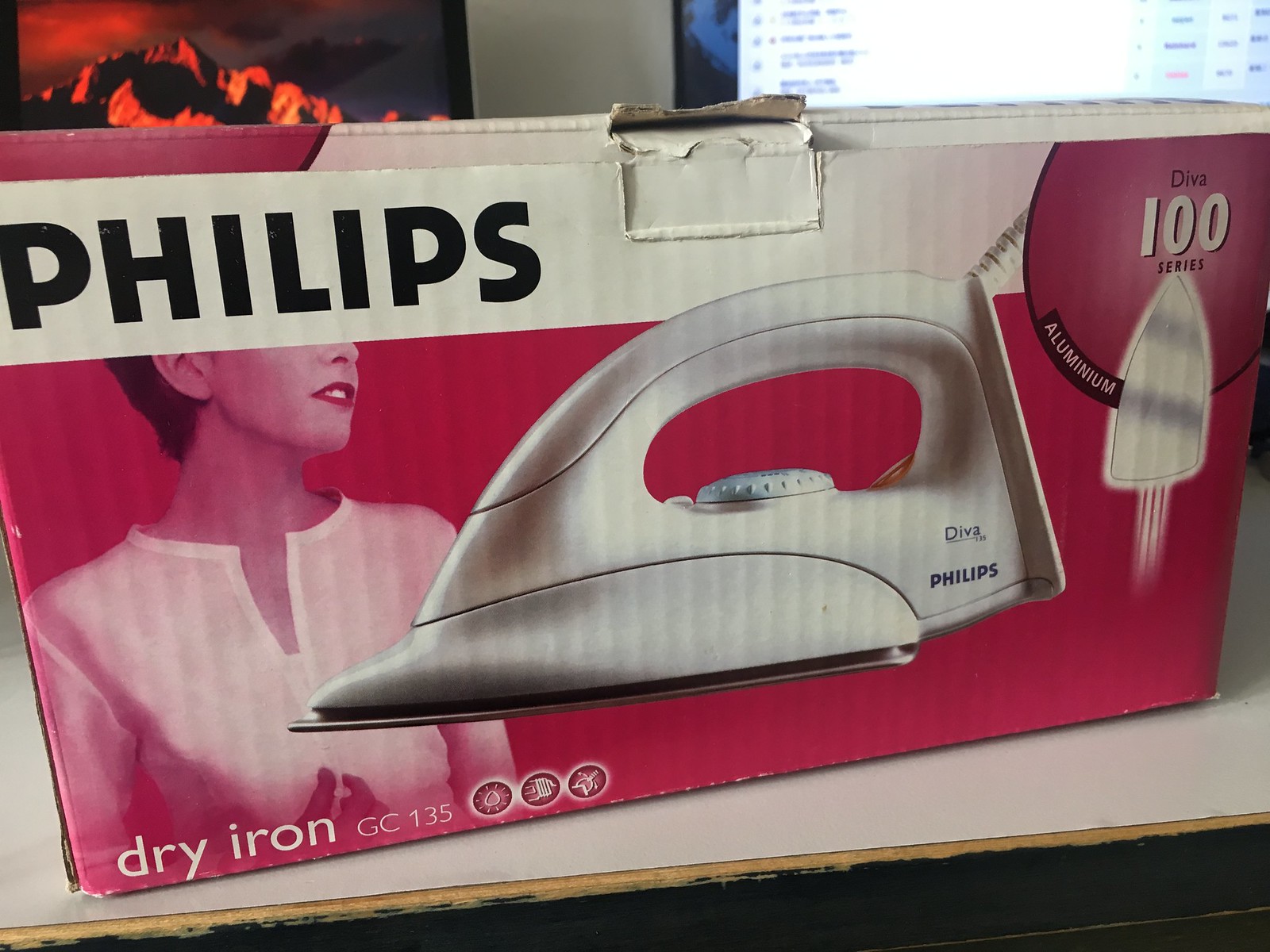This image features a detailed view of a cardboard box for a Phillips dry iron, specifically the aluminum GC135 model from the Diva 100 series. The box predominantly displays Phillips branding on the upper left corner, which appears faded. Initially designed to be a bright red, it now shows a more muted shade. The centerpiece of the box is an image of the silver iron itself, which appears almost three-dimensional. To the left, there's an image of a woman, cut off from the eyes up, wearing a white blouse. The edges of the box are noticeably ruffled, indicating that it has been previously opened. Behind the box, you can glimpse a computer monitor with a gray rim displaying a webpage, and another monitor in the background showing a mountain scene bathed in golden light. Additionally, the box features three symbols denoting the iron’s functionalities, though the details of these symbols are unclear.